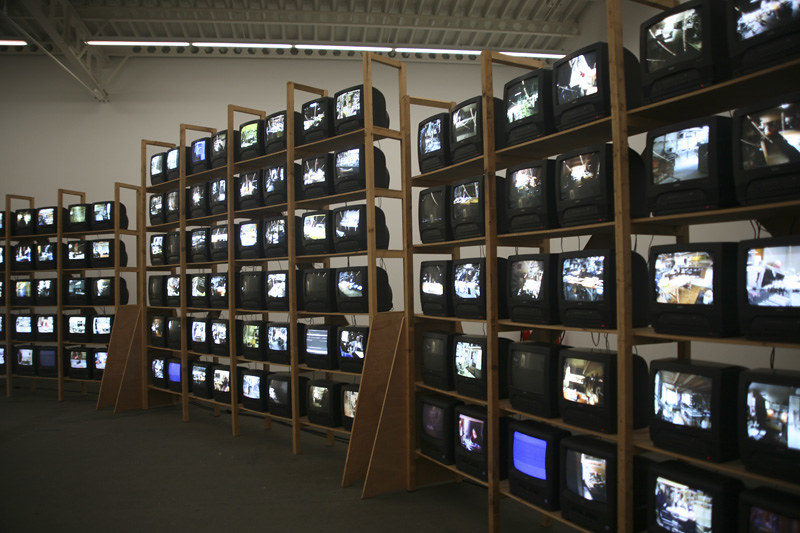This photograph captures the interior of what appears to be a large, open warehouse filled with old-fashioned CRT monitors. The scene is dominated by three expansive wooden shelving units, each ascending up to five or six tiers high, spanning horizontally across the room and exhibiting a slight curve from the right side to the left.

Each shelf supports two TVs per section, separated by middle posts, creating neat groupings of screens that are approximately 12 to 16 inches each. The middle shelf is particularly striking with its six-tier height and eight TVs per tier, totaling 48 screens. Adjacent shelves measure five rows high, each supporting four to six TVs per row.

A striking feature of this warehouse is its ceiling, lined with grid-like beams and fluorescent tube lighting that stretches into the distance, bathing the room in an industrial glow. The ground and walls are variations of gray, with the ceiling beams adding a stark contrast.

Every TV is operational, displaying an array of different scenes ranging from bright blue fuzz to static and images that resemble security footage of storefronts and interiors. This plethora of screens, their varied visual outputs, and the sheer number — estimated at over 100 units — create a visually arresting and slightly chaotic environment. Overall, the image portrays an almost surreal landscape of glowing monitors, each contributing a fragment to the visual cacophony within this expansive warehouse setting.